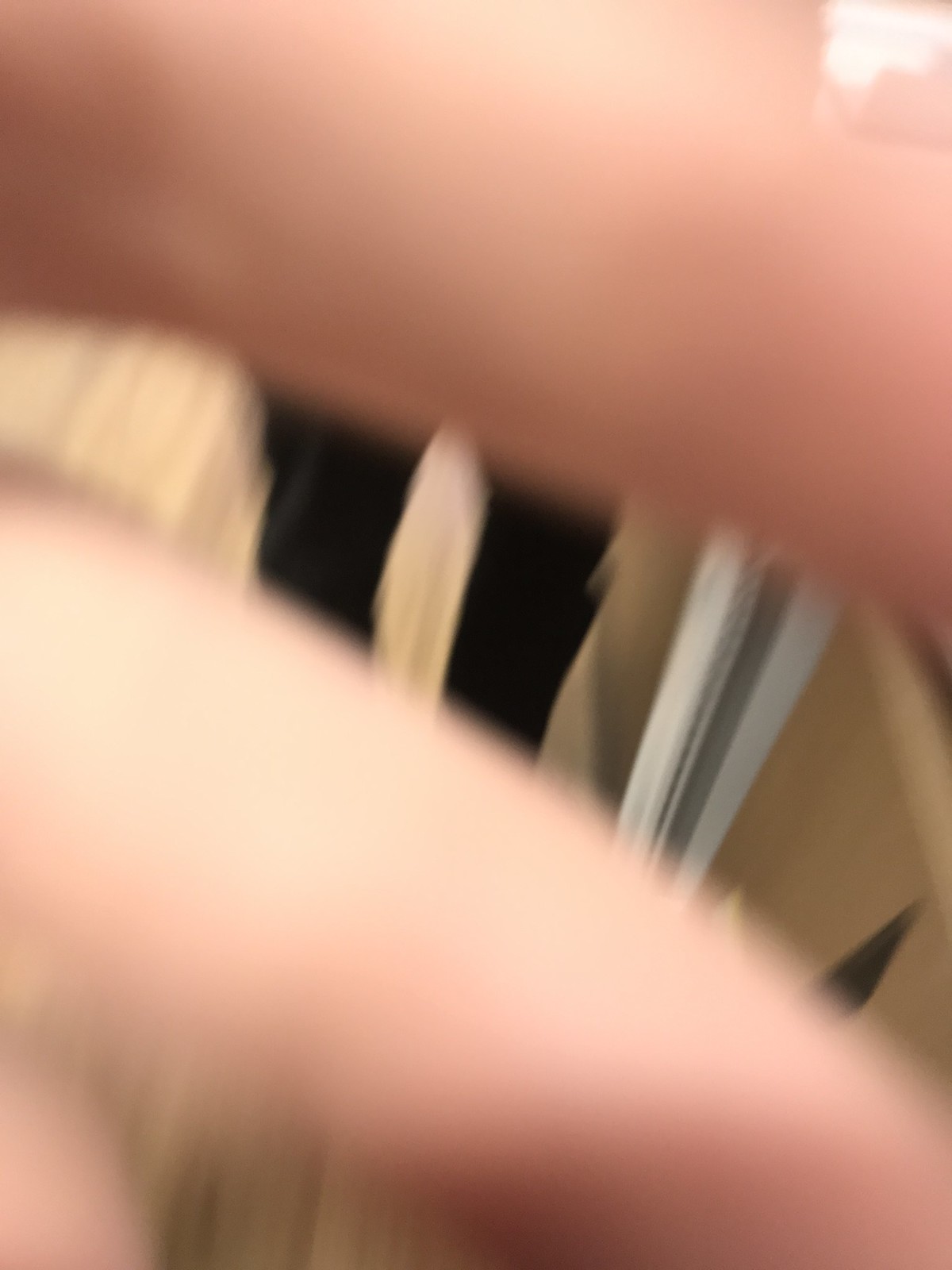The photograph shows a highly distorted and blurry image with what appears to be human skin, likely fingers, partially obscuring the lens. The image captures a scene that is difficult to make out but gives glimpses of a room or objects within it. Towards the bottom left corner and middle left side of the image, light-complexioned fingers are visible, with another finger extending from the top left to the top right corner. These fingers create a frame through which a cluttered and variably lit scene can be observed. 

The scene in between the fingers includes glimpses of several areas with different textures and colors; a wooden surface and various darker and lighter sections that alternate in a pattern, potentially indicating different materials such as carpet, furniture, or perhaps even notebooks or files. The left side of the image seems to have a sequence of beige, black, and other colors, while the right side features several areas resembling furniture in various shades like white, brown, and beige. The room itself appears brightly lit, without noticeable darkness, but everything within it is significantly out of focus and distorted, making specific details ambiguous.